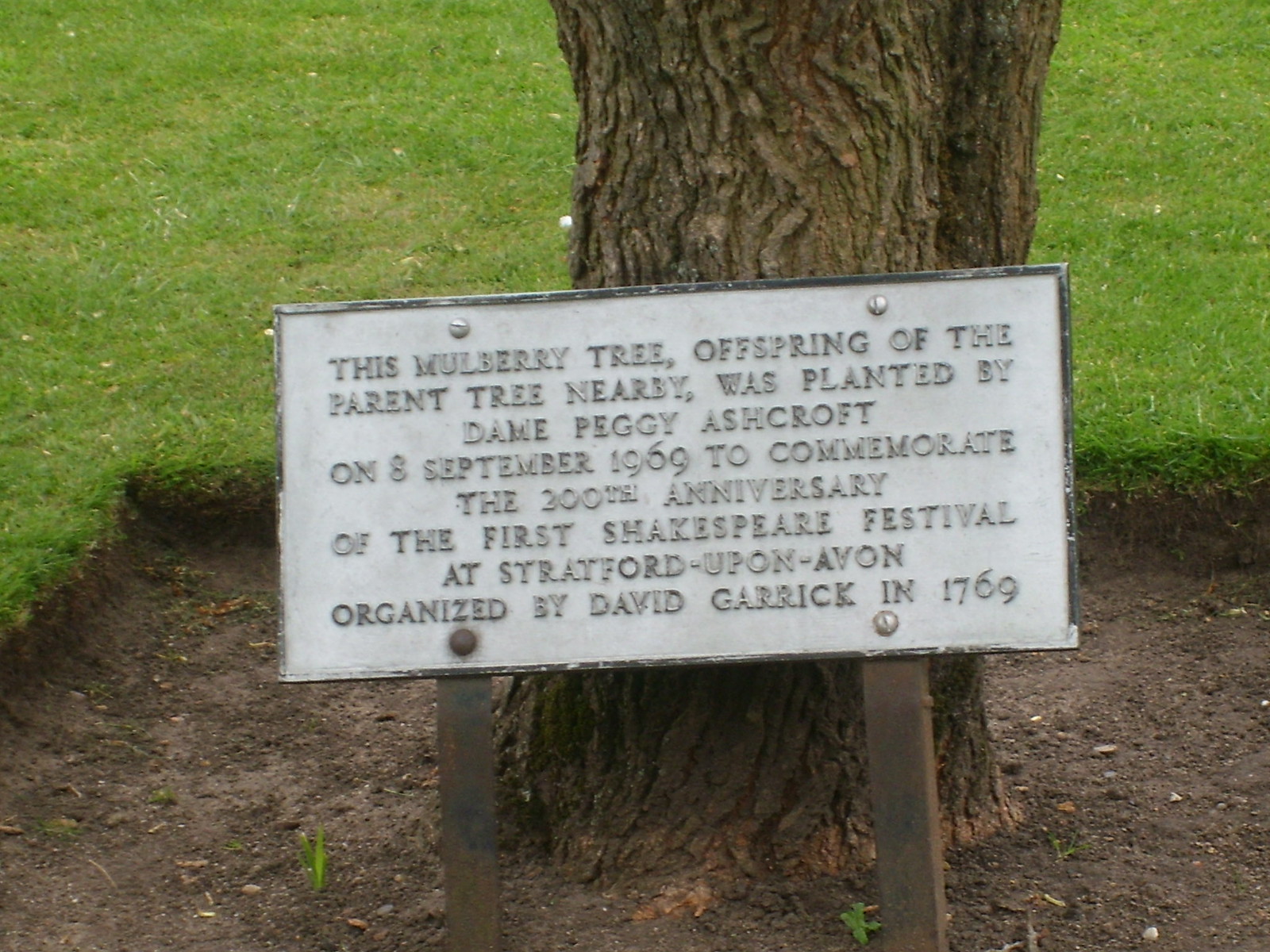The outdoor photograph showcases a scene dominated by a wide and robust tree trunk, encircled by a carefully maintained square patch of brown dirt. In the background, vibrant, dense green grass cut short adds a lush feel to the landscape. Positioned into the earth in front of the tree is an aged, gray metal sign with embossed lettering. The sign, although showing signs of wear and some scratches, reads: "This mulberry tree, offspring of the parent tree nearby, was planted by Dame Peggy Ashcroft on 8th September 1969 to commemorate the 200th anniversary of the first Shakespeare Festival at Stratford-upon-Avon, organized by David Garrick in 1769."